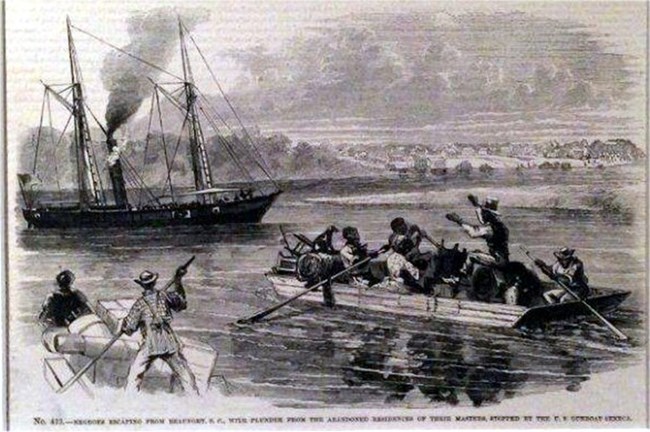A black and white illustration features a wide rectangular composition depicting a vivid scene on a large waterway. In the foreground, there are two smaller wooden rowboats: one carrying packages with two occupants—one steering and one passenger—and the second boat holding five African-American individuals rowing under the direction of a man standing in the center, arms outstretched. To the left side, a larger steamboat, characterized by tall steam stacks, masts, and numerous ropes, looms over the smaller vessels. The steamboat's deck is populated with troops, and crates and barrels are visible. The background showcases a sprawling landscape with an island lined with trees, a few houses, and a clearing. Above the town on the right side are ominous storm clouds, painted black with white outlines. The image is set against a cream or white backdrop marked by faint horizontal lines, and at the very bottom, there's a small, blurry, partially legible inscription that reads "N.O. 423."